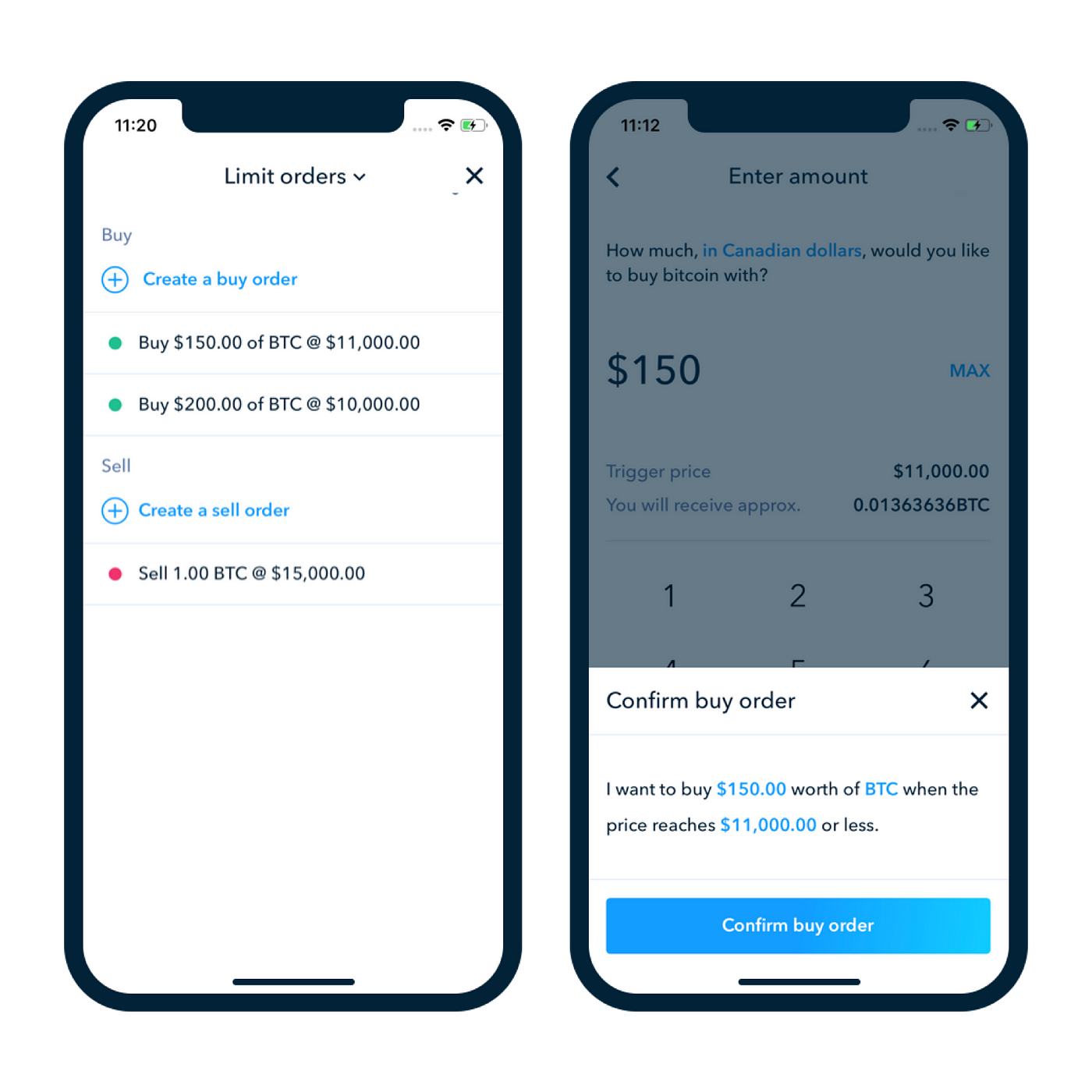**Descriptive Caption:**

On the left side of the screen, a trading interface is displayed with a clean, white background. The top section shows the current time, "11:20," in black text. Below the time, the heading "Limit Orders" is prominently displayed. 

The first section under the heading shows a blue button labeled "Buy." Immediately beneath, the text "Created Buy Order" is noted, followed by a thin gray line. Two green circles signify active buy orders. The first circle shows "Buy" with the amount "150.00 BTC" at a price of "$11,000.00." A second thin gray line separates this from the next order, which lists "Buy" with the amount "200.00 BTC" at a price of "$10,000.00." Another thin gray line follows. Below, a blue text indicates "Create a Sell Order," another thin gray line appears, and in red, it is noted: "Sell 1.00 BTC at $15,000.00."

On the right side of the screen, a confirmation pop-up is visible at the bottom. This pop-up features a white background with the heading "Confirm Buy Order" in black text. An 'X' is located in the upper right corner of the pop-up. Underneath, black text states "I want to buy," followed by the blue text "$100.00" and then black text "worth of." The word "BTC" is in blue, followed by "when the price reaches $11,000.00 or less," also in blue. 

A blue-bordered button at the bottom of the pop-up reads "Confirm Buy Order." Above this button, the text "Enter how much in Canadian dollars you would like to buy Bitcoin with" is displayed. The specified amount is "$150" and the max trigger price is set to "$11,000.00," indicating that approximately "0.01363636 BTC" will be received upon execution of the order.